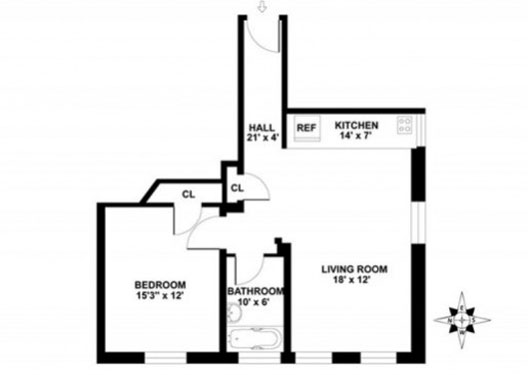Detailed Blueprint Description for a One-Bedroom House:

This image showcases the detailed blueprints of a compact, yet well-planned one-bedroom house. As depicted, the house features a small yet practical kitchen, measuring 14 feet in length and 7 feet in width. The kitchen is efficiently laid out with the refrigerator located at one end and the cooktop at the opposite end.

Attached to this cozy culinary space is a spacious 18-by-12-foot living room, providing a comfortable area for relaxation and entertainment. Adjacent to the living room, there's a narrow hallway that spans 21 feet long and 4 feet wide, likely serving as a passage from the front entrance into the main living areas.

The bedroom, which is quite sizeable, measures 15 feet, 3 inches by 12 feet, offering ample space for furniture and personal belongings. Complementing the bedroom, there are two closets in the house: a dedicated bedroom closet and an additional coat closet conveniently placed near the entrance for guests and residents.

Positioned strategically between the living room and the bedroom, the bathroom spans 10 feet by 6 feet. It features a combined shower tub, a sink, and a toilet, ensuring all the necessary amenities are within easy reach. Notably, the bathroom is situated on the opposite side of the house from the kitchen, enhancing privacy and accessibility.

Overall, this well-thought-out one-bedroom house blueprint demonstrates both functionality and efficient use of space, making it a highly livable and inviting home.